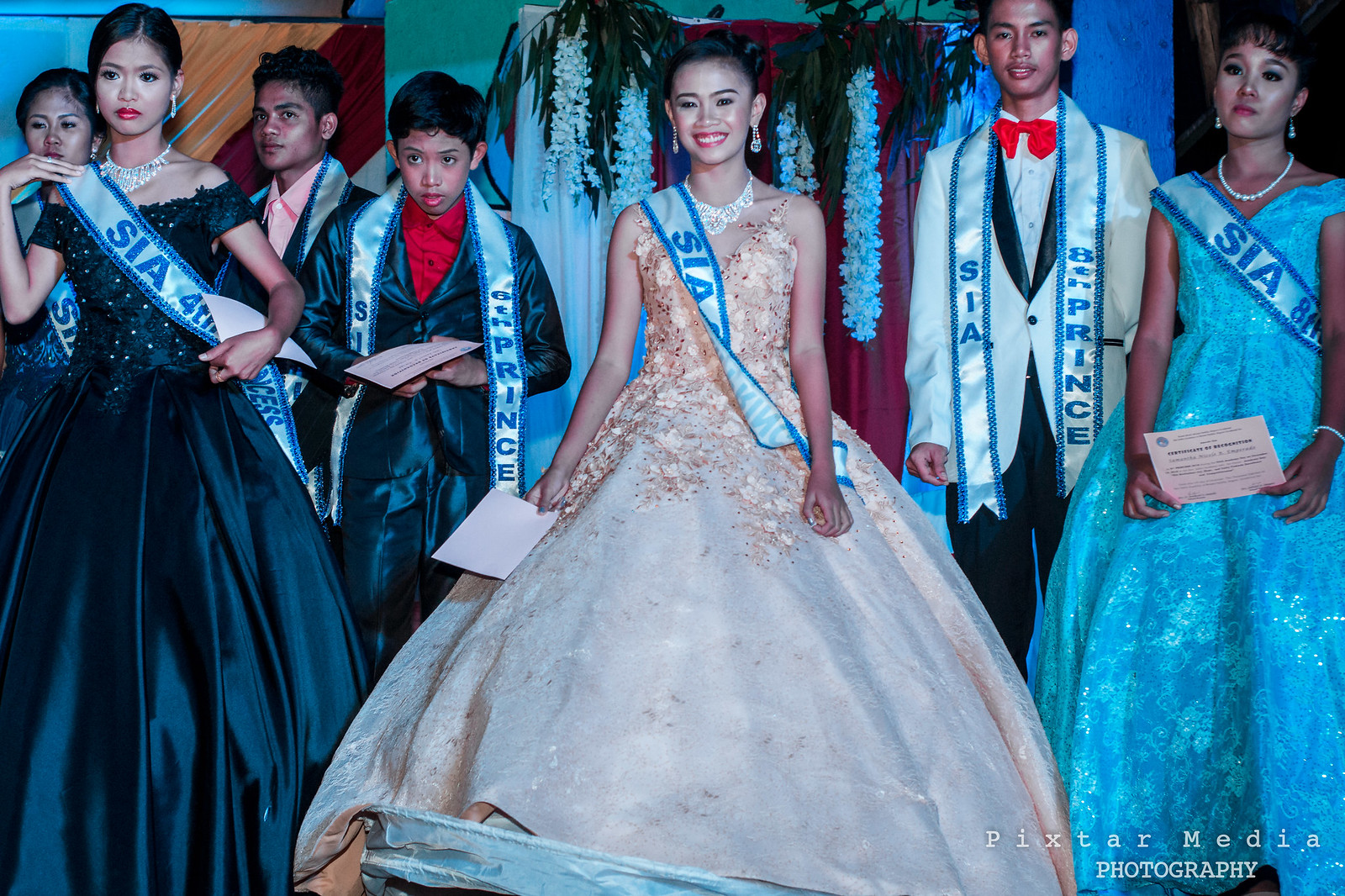In this image, several young people are dressed in elaborate attire, reminiscent of a pageant or formal dance. Centrally featured is a woman wearing a lavish ball gown that flares out from the waist, adorned with large sequins on the cream-colored bodice. Her hair is elegantly pulled back, and she's accessorized with a sparkling bracelet, earrings, and a necklace. A white sash with a blue border drapes over her shoulder, displaying the acronym "S.I.A." and she holds a piece of paper in one hand, smiling radiantly. Surrounding her are other contestants, split evenly between males and females. The females are in vibrant ball gowns of various colors, including peach, light blue, and black, with intricate lace and applique details, while the males don sophisticated, colorful tuxedos and suits, featuring materials like satin, one with a shiny blue jacket and another sporting a white vest with blue pants. Each contestant also wears a sash similar to the central woman's, with additional inscriptions like "Prince" followed by different numbers. The group appears somewhat disinterested or somber, with only a few faint smiles scattered among them. In the background, there are more contestants and decor elements such as leis and curtains, adding to the festive atmosphere of the scene. The bottom right corner of the image is marked with "Pixar Media Photography."